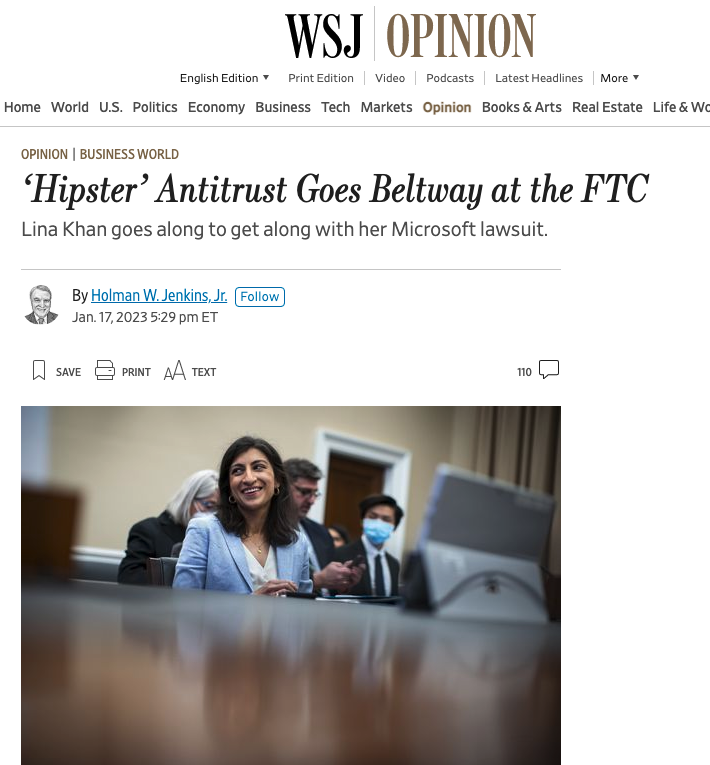**Image Caption:**

A screenshot from the Wall Street Journal's Opinion section dated January 17, 2023, at 5:29 PM EST, features an article titled "Hipster Antitrust Goes Beltway at the FTC" with the subtitle "Lena Khan Goes Along to Get Along with Her Microsoft Lawsuit," authored by Holman W. Jenkins, Jr. The article falls under the Opinion, Business World subheading. The screenshot includes interactive icons for saving, printing, and adjusting text size, and indicates there are 110 comments on the piece. The image shows Lena Khan, the FTC Chair, likely in a formal setting such as a meeting or hearing, smiling and looking to the side. She is wearing a light blue blazer. The background shows other individuals, some wearing face masks, along with various pieces of equipment. Above the article, the website navigation bar lists sections such as Home, World, U.S., Politics, Economy, Business, Tech, Markets, Opinion, Books & Arts, Real Estate, and Life & Work. The article discusses Lena Khan's approach to antitrust enforcement, focusing on a lawsuit involving Microsoft.